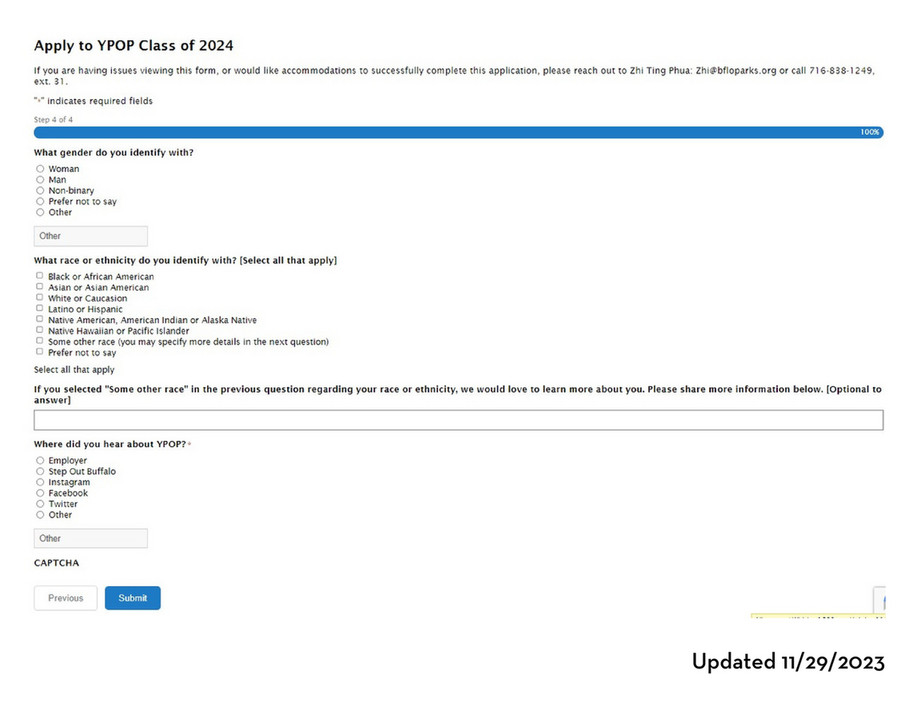**Apply Now: YPOP Class of 2024**

The website showcases the application form for the YPOP Class of 2024, with a recent update noted at the bottom, dated November 29, 2023. Just above this update, there's a small yellow icon that seems to indicate the start of another section of the page.

There is an accessibility notice for users experiencing difficulties with the form or requiring accommodations to complete it, directing them to contact Zhiting Fu via the provided email and phone number, including an extension. Required fields are indicated with an asterisk.

The form is on the fourth and final step, confirming this is the end of the questionnaire. It begins by asking, “What gender do you identify with?” with options: Woman, Man, Non-Binary, Prefer not to Say, and Other.

Following this is a question about racial or ethnic identity with a directive to select all applicable options. The choices include:
- Black or African American
- Asian or Asian American
- White or Caucasian
- Latino or Hispanic
- Native American, Native Indian, or Alaskan
- Native Hawaiian or Pacific Islander
- Some Other Race
- Prefer Not to Say

The next question invites applicants who selected “Some Other Race” to provide additional details, though this response is optional.

Subsequently, the form inquires, "Where did you hear about YPOP?" listing options such as Employers, Step Out Buffalo, Instagram, Facebook, Twitter, and Other.

The form concludes with navigation buttons for “Previous” and “Submit,” and likely includes a CAPTCHA verification to proceed.